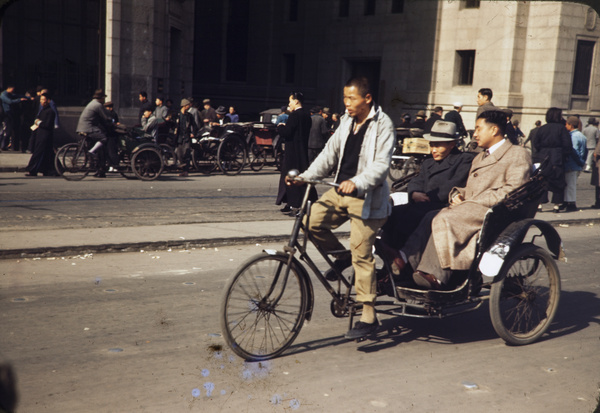In this angled photograph, we see a classic bicycle taxi in what appears to be an Asian country, distinguished by its rusted frame and thin front wheel. The driver, dressed in a grey jacket over a black shirt, tan pants, and black shoes, pedals diligently down a littered street. The black carriage attached to the back carries two well-dressed passengers. The man on the left dons a long black coat and a grey hat, engrossed in reading a paper, while the man on the right, sporting a long brown trench coat over a white button-up shirt and tie, peers at the same paper. Both have an air of refinement, with the latter man wearing his short black hair neatly. Surrounding them, other bicycle taxis and pedestrians populate the scene, with a large stone white building visible in the background. The overall atmosphere suggests this photograph, likely from the 60s or 70s, captures a moment in the daily hustle and bustle of the city.